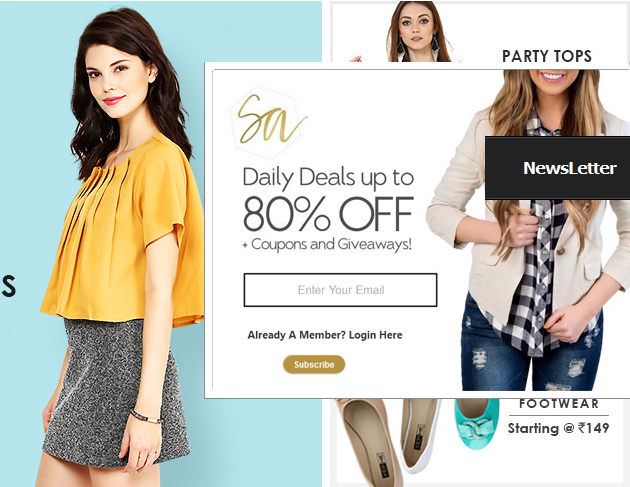This is a detailed description of a screenshot from the SA Clothing website, showcasing a split image—each side offering different visual content, overlaid by an email solicitation pop-up box.

On the left side, there's a photo of a model standing against a blue background. The image is cropped, showing part of an 'S' on the center-left, indicating that some text was cut off in the process. The model appears to be center-stage, but due to the cropping, only part of the scene is visible.

The right side of the split image focuses on different products available from the website. A model is positioned at the top left, and the words "Party Tops" are displayed towards the right. However, the pop-up box obstructs some of the content on this side.

The pop-up, with a white background, is overlaid through the center of both images. At the top left corner of the pop-up is the SA logo, displayed in gold letters inside an octagon. Below the logo, the text reads "Daily Deals up to 80% off plus coupons and giveaways." The next line invites users to "Enter your email" for further engagement. There is also a prompt for existing members to log in, indicated by the phrase "Already a member? Log in here." To the right of this text, a gold 'Subscribe' button is prominently displayed.

Additionally, there is a black box located towards the center-right of the pop-up, containing the word "Newsletter" in white letters, reinforcing the invitation for users to subscribe to ongoing deals and information updates from the SA Clothing website.